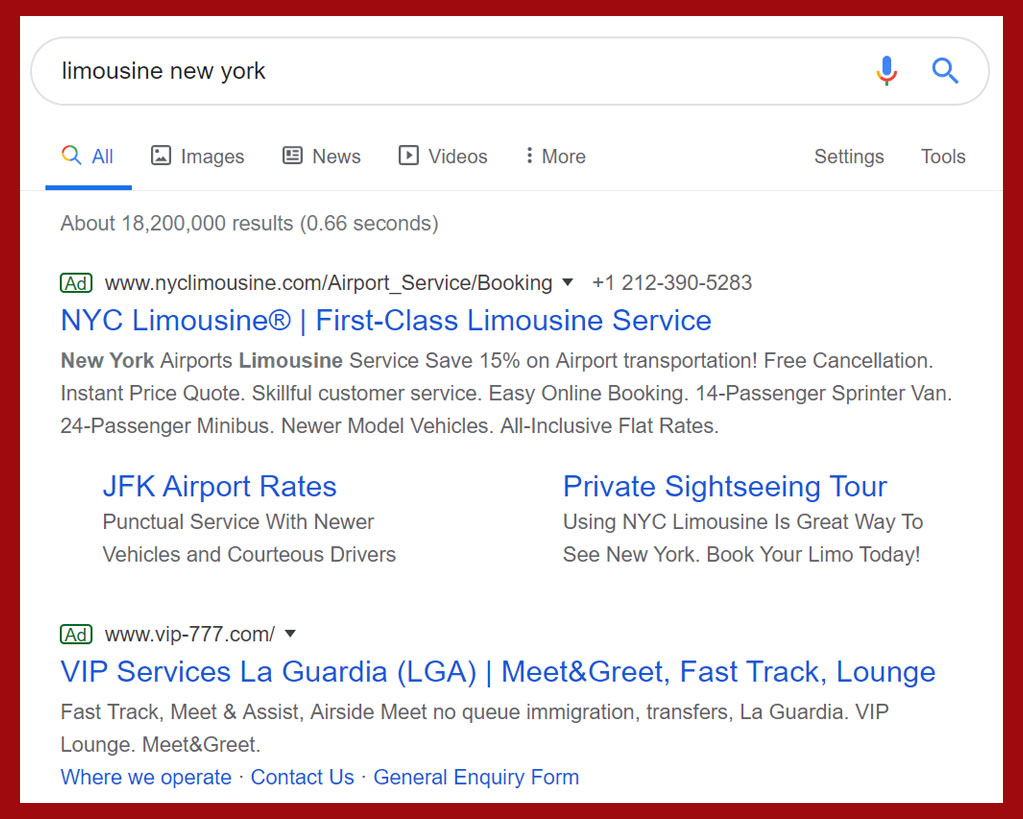This image features a screenshot with a prominent red rectangular border surrounding a white background. At the top of the screenshot, a search bar contains the dark gray text "Limousine New York," accompanied by the Google microphone icon and the Google magnifying glass icon to the right. Directly below the search bar, a navigation menu spans from left to right, displaying options labeled “All,” “Images,” “News,” “Videos,” “More,” “Settings,” and “Tools.” The "All" option is highlighted in blue, indicating it is the currently selected category.

In the main content area below the menu, there's a visible URL in blue text, "www.nyclimousine.com/airport_service/booking," followed by a contact number, "1-212-390-5283," also in large blue text. Directly underneath this, the headline "New York City Limousine: First-Class Limousine Service" is prominently displayed. The advertisement contains additional links in blue text, with “JFK Airport Rates” positioned to the left and “Private Sightseeing Tour” to the right.